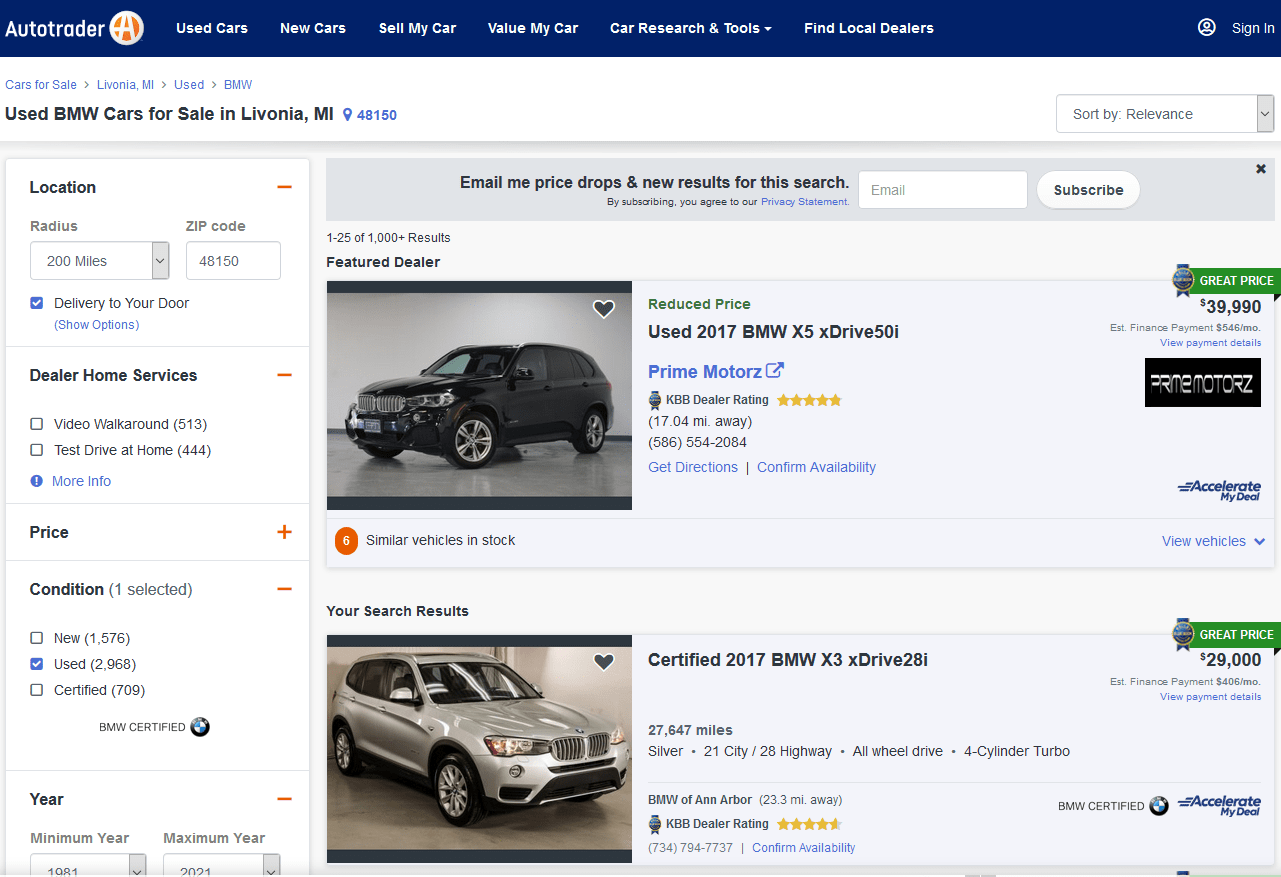This is a screenshot from the Autotrader homepage. The top border is dark blue, adorned with the Autotrader logo in the left corner—a white "Autotrader" text accompanied by an orange circle featuring a white "A" with a white border. Moving from left to right, the navigation menu includes options: "Used Cars," "New Cars," "Sell My Car," "Value My Car," "Car & Research Tools," and "Find Local Dealers." On the far right, there is a sign-in option with a profile icon next to it.

Below the top border, about an inch of white space is bordered in blue with small text reading "Cars for Sale." Below, larger black text spells out "Used BMW Cars for Sale in Livonia, MI," and a blue location pin denotes the zip code 48180. The right side of this section contains a search bar labeled "Sort by Relevance."

On the left side of the page, a white rectangle occupies about a third of the way across, extending below the screen's bottom. This section includes a "Location" header with two location tabs, one featuring a blue checkmark and the option "Deliver to your door." Below, the bold black text "Diller Herms Services" is followed by related information marked with white squares and black borders.

Further down, bold black text displays "Plot Price" with a plus sign on its right. Next, a section labeled "Condition" includes a minus sign, with checkboxes for "New," "Used," and "Certified." The "Used" option is checked, marked by a blue square with a white checkmark, and below it reads "BMW Certified."

To the right, black text prompts users to "Email my price drops and new results to this search," accompanied by an email input field. Underneath this are two search results, each displaying a car on the left, detailed information in the center, and another view of the car on the right.